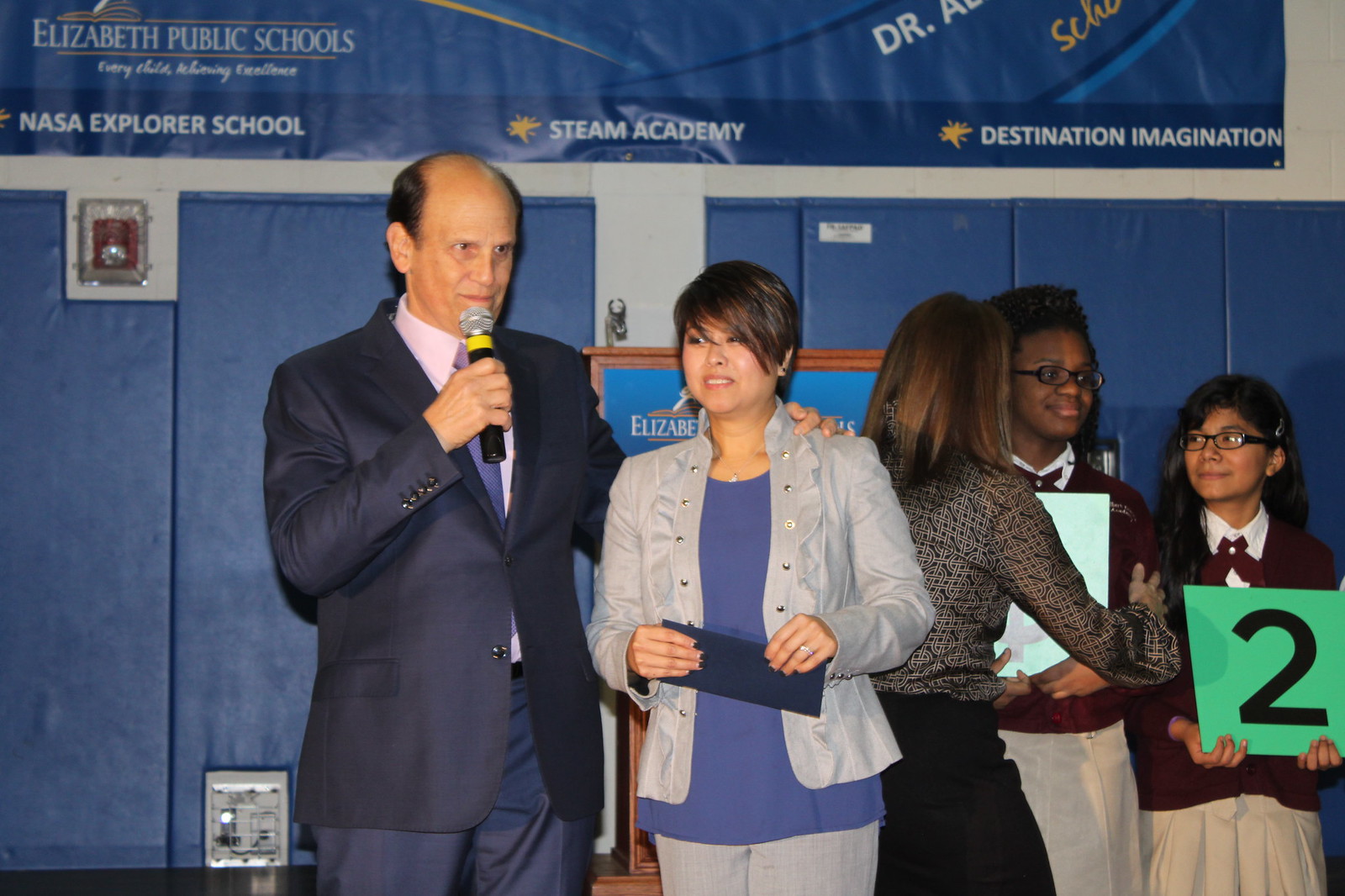The image captures a moment on stage indoors, featuring two people in focus. An older man, balding on top but with ample hair on the sides, is holding a microphone with a silver top, yellow band, and black handle. He is attired in a dark suit comprising a black blazer over a pink or light purple button-down shirt, paired with a blue tie and dark pants. His arm is affectionately around the shoulder of a woman with short, ear-length, black hair with brown highlights, who is dressed in a blue shirt beneath a gray or light blue ruffled jacket, and white or light gray pants. She holds a blue envelope or paperwork. Behind them are three additional individuals: a woman turned away, and two high school-aged girls in what appear to be school uniforms, perhaps holding posters, one of which bears the number two. They are standing in front of a blue padded wall, suggesting the setting is a gymnasium. Above them hangs a banner reading "Elizabeth Public Schools, NASA Explorer School, STEAM Academy, and Destination Imagination."